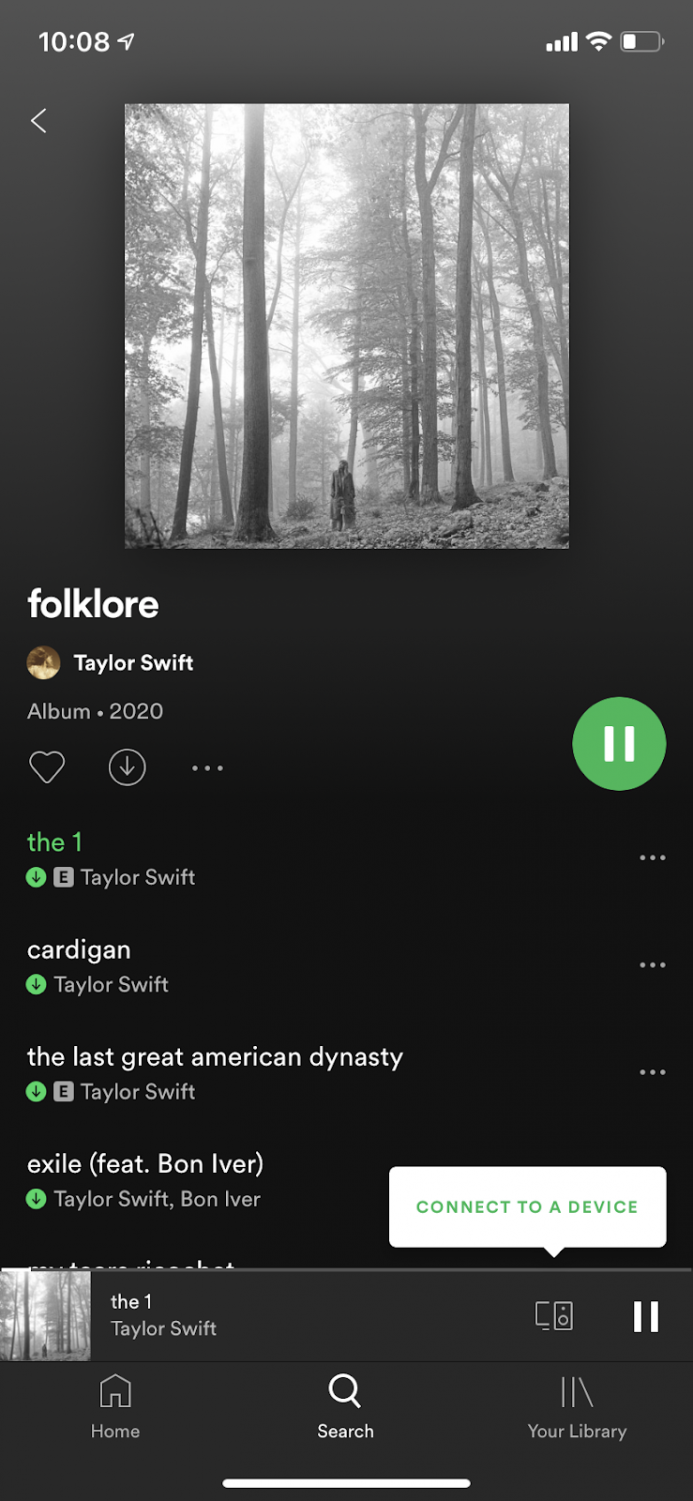A phone screenshot displays a Spotify interface. In the top left, the time reads 10:08, and in the top right, a battery icon shows 20% remaining alongside fully filled Wi-Fi and phone signal bars. The album cover, occupying the top half, features an image of a forest with tall trees, where a figure stands at the bottom center, gazing leftward. Beneath the artwork is the title "Folklore" and the artist's name, Taylor Swift, followed by the album designation and the release year, 2020. To the right, a green circle with a white plus symbol suggests adding the content to a collection. The bottom half lists four song titles: "The One," "Cardigan," "The Last Great American Dynasty," and "Exile (feat. Bon Iver)."